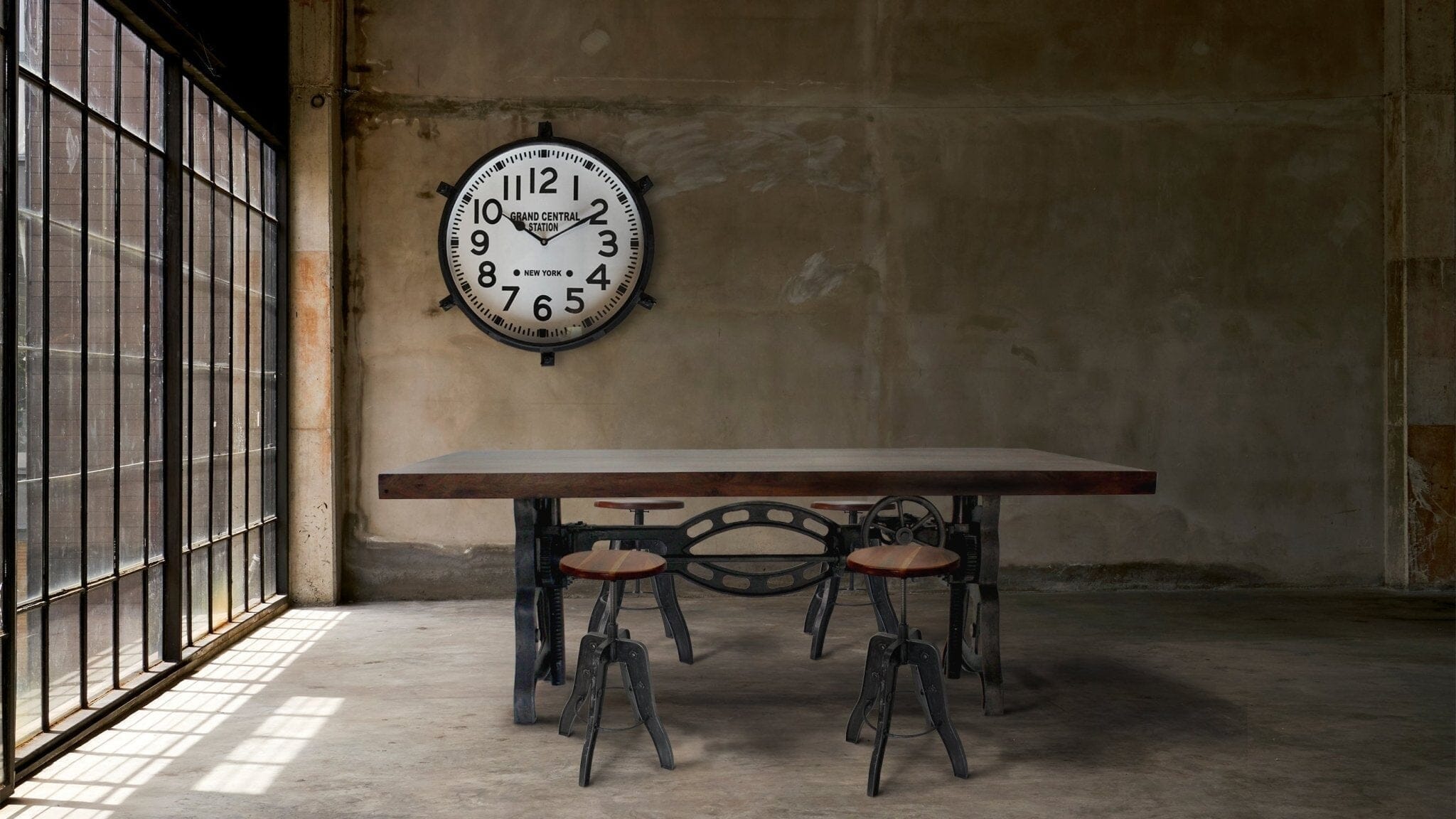The image depicts an industrial interior space within Grand Central Station, characterized by its stark concrete walls and floors. Dominating the room is a substantial wooden table with a thick top, supported by a heavy black cast iron or steel frame, accompanied by four matching stools. Positioned centrally, the table measures approximately 10 feet in length and 4 feet in width. To the left, there is a large window that spans the height of the room, divided into two sections and featuring vertical black bars spaced about four to five inches apart. Additionally, thinner horizontal lines run across it, giving the appearance of a sliding door. The room is sparsely decorated, with the only notable feature being a large, white-faced analog clock mounted on the wall. This clock, marked with bold black Arabic numbers from 1 to 12, reads 10:10 and bears the inscription "Grand Central Station." The overall ambiance is minimalist and utilitarian, with an emphasis on raw materials and functional design.